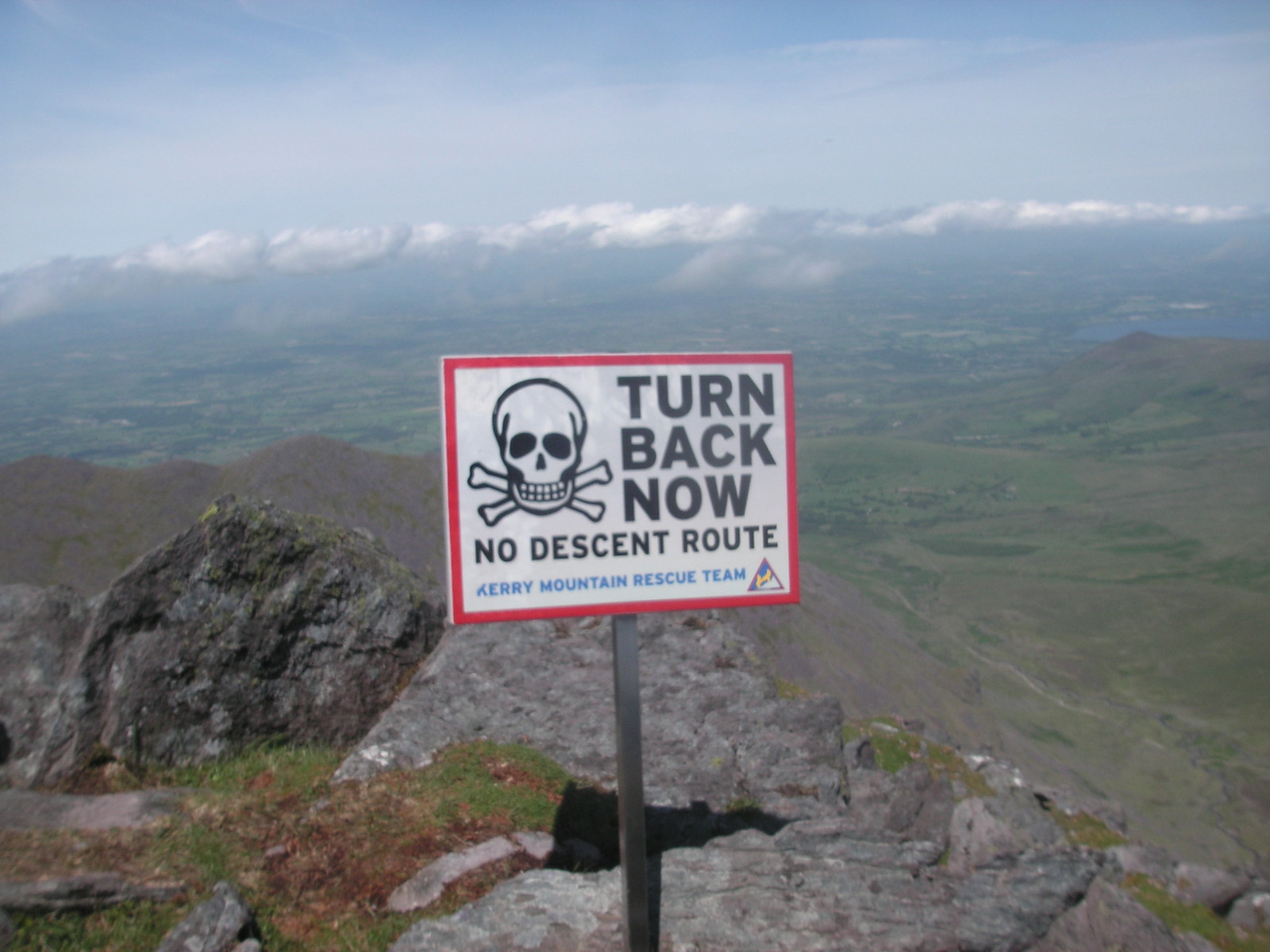The photograph captures a breathtaking view from the peak of a mountain, presenting an expansive and varied landscape. From this high vantage point, the scene unfolds with lush green forests and sprawling fields stretching towards the horizon. The area below is vast and diverse, featuring patches of dirt and blue water bodies on both the left and right sides. Near the bottom of the image, a rugged cliff adorned with brown rocks, patches of green grass, and dirt is prominently visible.

The sky above is a striking bluish-gray, interspersed with feathery white clouds that seem to brush the mountain tops, creating a surreal feeling of being at cloud level. In the distance, a body of water glimmers, adding to the serene yet wild beauty of the scene.

A notable element of the photograph is a prominently displayed warning sign mounted on a black post. The sign, bordered in attention-catching red, features a stark white background emblazoned with a black skull and crossbones. In bold black lettering, it reads: "Turn back now, no descent route." Beneath these foreboding words, in blue font, is the declaration "Cary Mountain Rescue Team," accompanied by what is assumed to be their logo—a triangle filled with blue, yellow, and white. The sign sternly warns of the dangerous terrain, underscoring the perilous nature of this majestic yet formidable location.